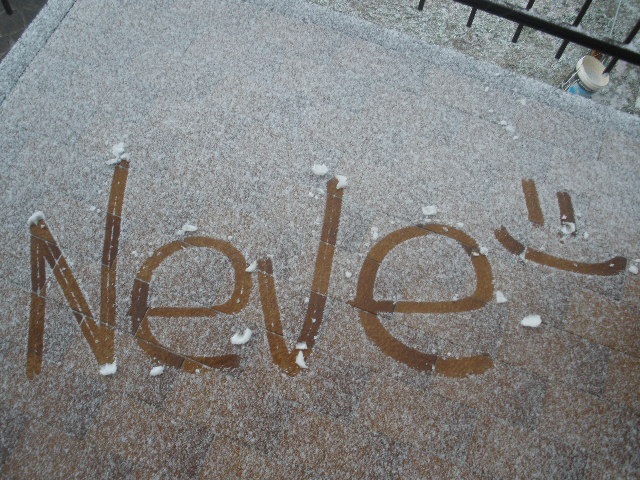This image captures a frosty scene on what appears to be a porch or possibly a balcony with a thin layer of snow dusting the wooden planks below. The snow is thin enough to still reveal the striations and texture of the wood beneath. In the upper right-hand corner, a black fence with vertical bars can be seen, providing a safety barrier typical for porches or balconies. The main focal point of the image is a message written in the snow: "NEVE," spelled in capital letters, followed by a simple smiley face composed of two lines and a half-circle. The snow also partially covers a nearby area, where a brownish, stone-like texture is visible, possibly indicating a transition between different flooring materials. Additionally, a discarded fast food cup lies on the ground, contributing to the scene's sense of casual, everyday life amidst the wintry setting.